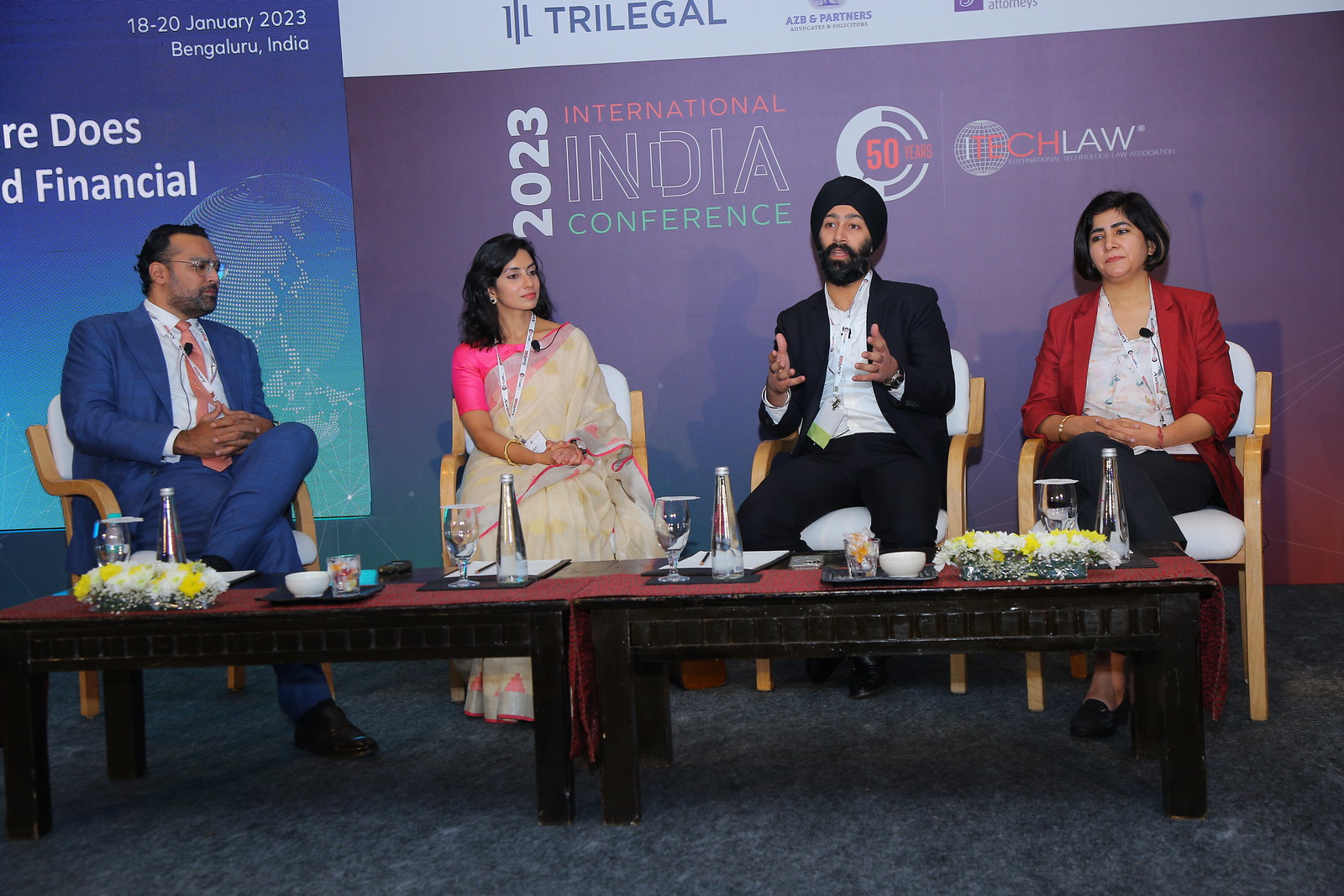The image captures a vibrant scene at the 2023 International India Conference held from January 18th to 20th in Bengaluru, India. Four individuals of Indian descent are seated at a low conference table covered with a red tablecloth, adorned with white and yellow flowers, clear bottles, and glasses. From left to right, the first person is a man, approximately 45 years old, in a blue suit with an orange tie and glasses. Next to him is a woman in her early 30s, donning a beige sari paired with a pink blouse. To her right sits a man distinguished by his black turban, black suit, black beard, and white shirt. The rightmost individual is a woman dressed in a red sports coat over a white shirt paired with dark pants. They are positioned against a backdrop featuring a prominent purple sign that reads "2023 International India Conference, 50 years, I-tech law," signifying the event’s theme and location. The overall style of the photograph is realistic, depicting a conference discussion in progress.